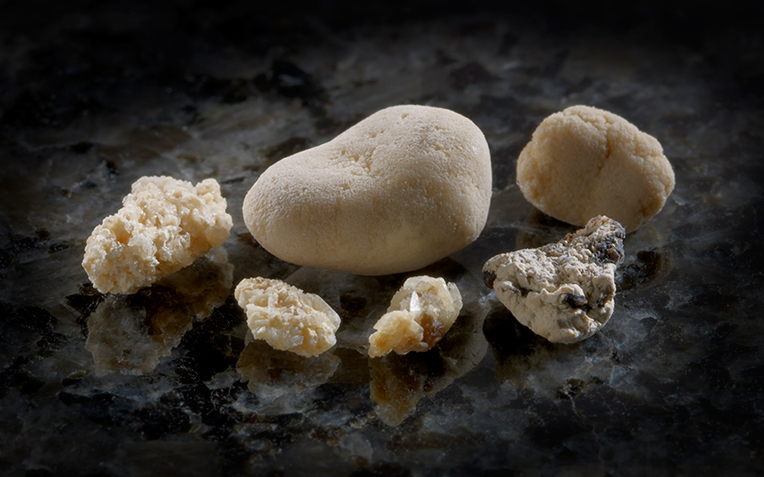This detailed photograph captures an assortment of six beige and white rocks, arranged on a flat, black, and likely granite or marble surface, with a focused light illuminating them. At the center of the arrangement, the largest rock resembles a white potato, smooth with some skin pitting, wider at the top right and tapering to a dip at the bottom left. To its left, there's a yellowish, chunky rock with many nooks and crannies, evoking the look of melted ears of corn or popcorn. Nearby, another smaller rock shares this rough, popcorn-like texture. On the right side of the central rock, there are two more similarly textured rocks, with the first being a bit lighter in color and the second showing a smoother appearance with black flecks. Further right, there’s a rock that looks like a broken piece of a larger stone, revealing gray and black interior surfaces. Completing the array is an oval, sponge-like rock with a brownish tint and a surface full of tiny holes, akin to cauliflower. The indoor setting allows for the intricate details of each rock to be highlighted against the shiny, dark background.